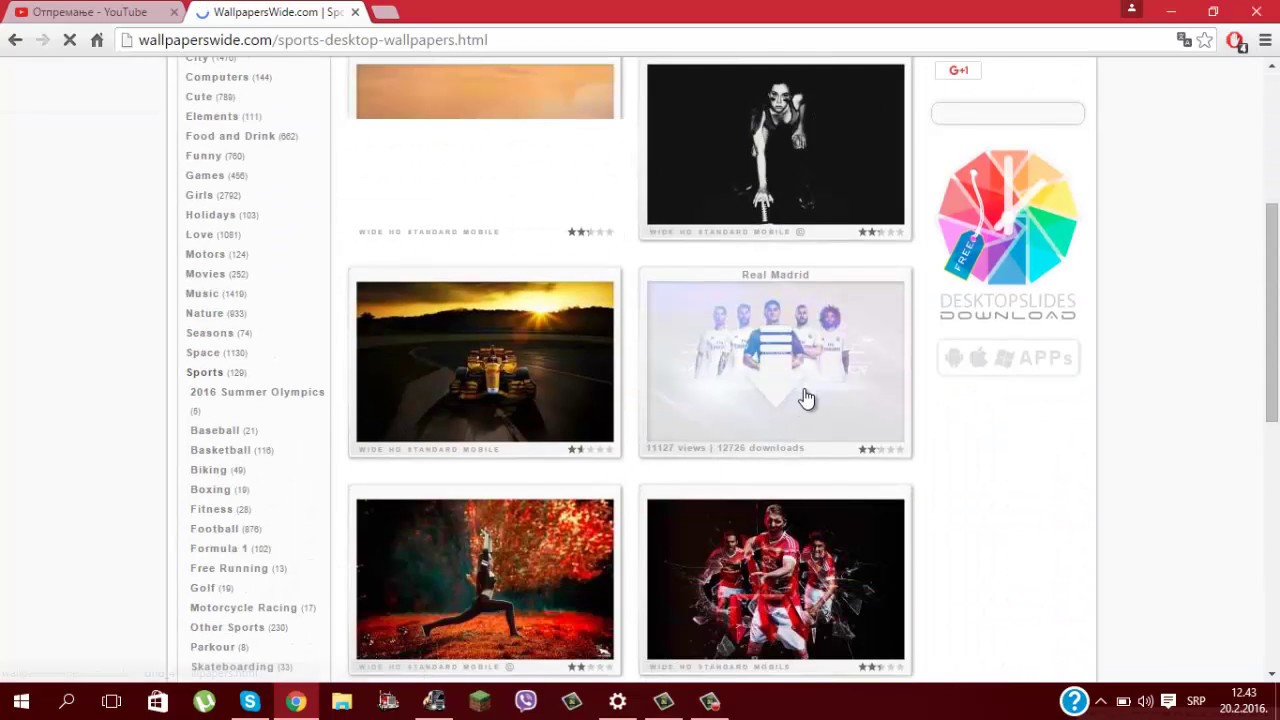In this screenshot from the website WallpapersWide.com, a user is browsing through various wide-format wallpapers for their desktop. The focus is on the "Sports" category, which is highlighted on the left side of the screen. The available options within this category include several images related to different sports events and activities. Specific wallpapers visible include an image from the 2016 Summer Olympics, a Formula One racing scene, a dynamic long jump over a field of red grass with a striking red tree in the background, and a group photograph of footballers posing together. The user is not searching for any specific type of wallpaper but appears to be exploring the diverse selection available within the sports theme.